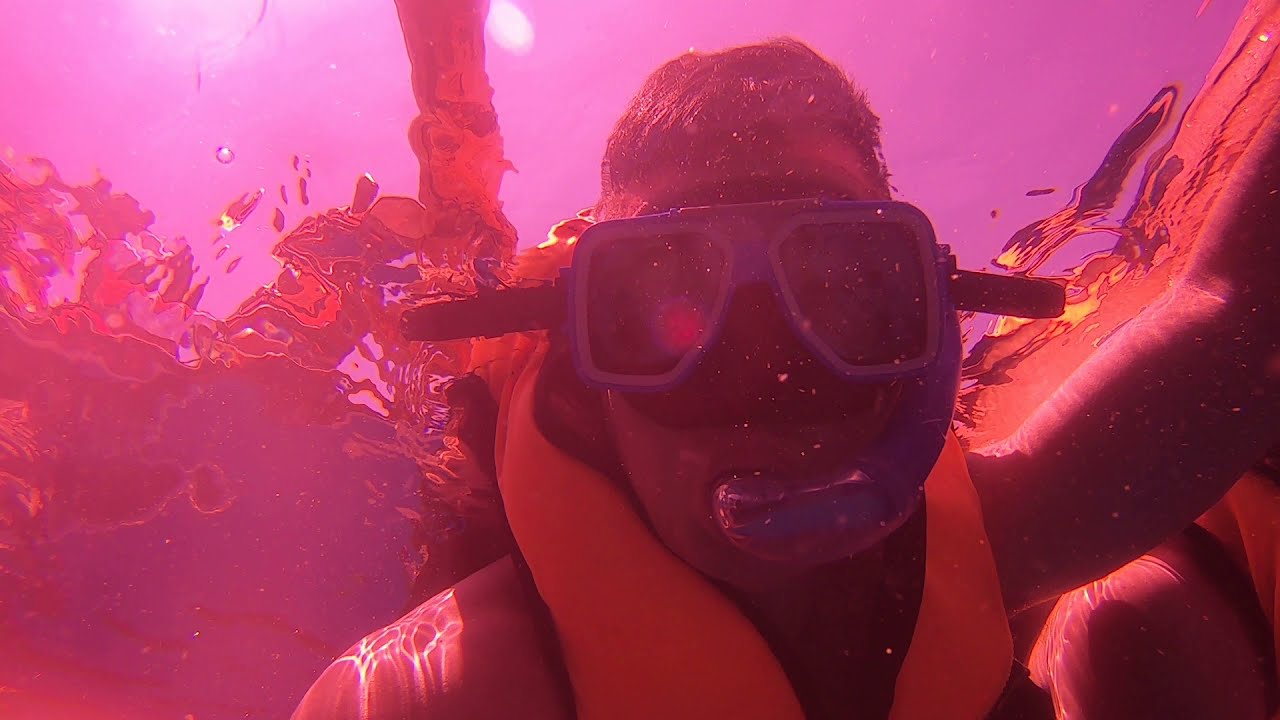This image features a man underwater, seemingly snorkeling, though there is some ambiguity as no tank or definitive snorkel is visible. The scene has an overall striking pink hue, suggesting a surreal or abstract quality, possibly staged. The man wears a purplish mask and a yellow diving vest over a black wetsuit. His right shoulder shows a water reflection, indicating submersion. The background depicts fish swimming, contributing to the aquatic setting. Light appears to come from the top left, enhancing the pink ambiance. Overall, this image blends elements of underwater exploration with an unusual and vibrant color palette.